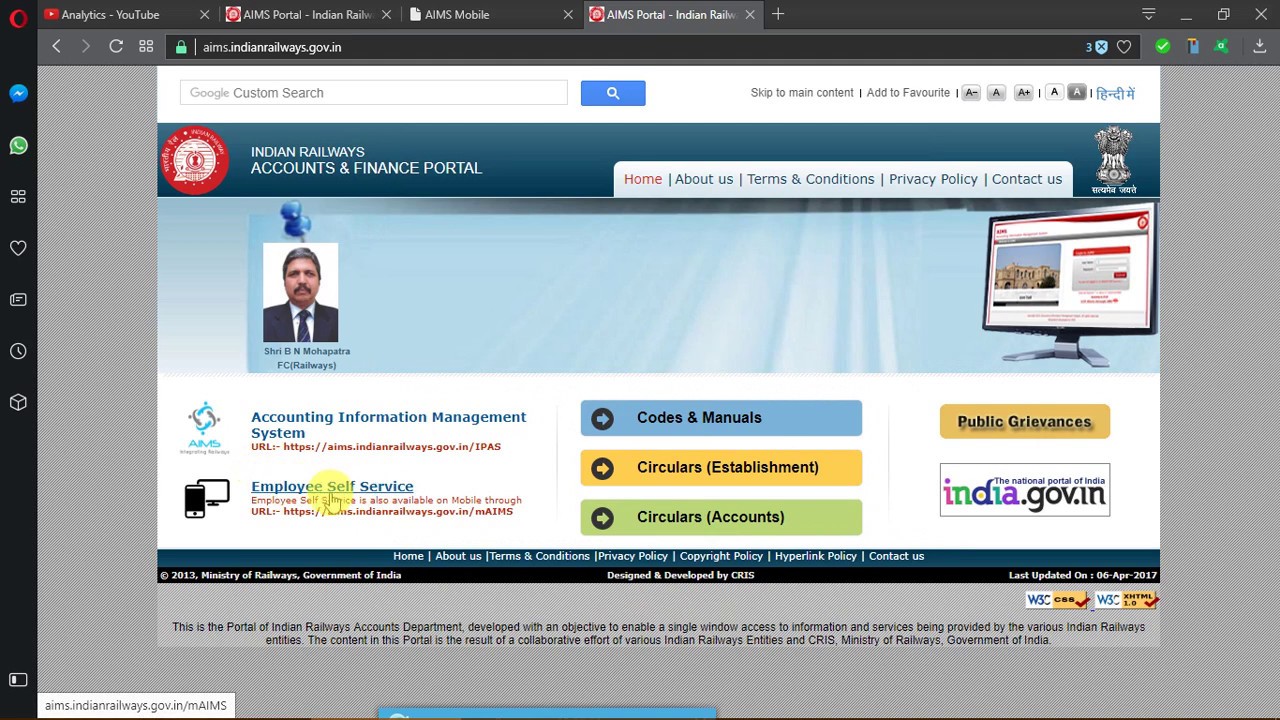The image is a detailed screenshot of a web portal, specifically tailored for the Indian Railways Accounts & Finance Portal.

The interface features a prominent black left and top border. The top of the page hosts a series of tabs with white text that are too small to discern and vertical icons lining the left side. The main section of the screen has a gray background with a white page overlay. At the top of this white page, a search bar labeled "Google Custom Search" is highlighted by a bright blue background and a white magnifying glass icon. 

Centered at the top left, a logo is depicted, consisting of a white circle with red framing and font. Adjacent to this, in capital letters, "INDIAN RAILWAYS" is written in white, followed by "Accounts & Finance Portal" on the next line. To the right, a menu lists several items: "Home" in red, followed by "About Us," "Terms and Conditions," "Privacy Policy," and "Contact Us" in dark font. An icon is situated to their right.

Below this, a light blue section contains an image of a man in a suit with a mustache, accompanied by a blue thumbtack icon above his head. Although his name is present beneath the image, it is illegible. On the far right, an image of a computer appears. Under it, the text "Accounting Information Management System" is written in blue, accompanied by an icon to the left. Beneath this, a brown URL is followed by "Employee Self-Service" highlighted in blue text and an accompanying icon. A partial thumbprint graphic in yellow overlies this section.

Central to the page, three horizontal rectangular panels are prominent. The first panel is blue with bold black text reading "Codes and Manuals." The second panel, with a yellow background, reads "Circulars" followed by "(Establishment)" in parentheses. The third panel has a green background with "Circulars" followed by "(Accounts)" in parentheses. Each panel is marked by a black circle icon with a right-pointing arrow. To their right, a button marked "Public Grievances" features black text on a yellow background. Below, a white box bordered in dark color reads "india.gov.in" in lowercase.

This detailed description outlines the comprehensive layout and design elements of the Indian Railways Accounts & Finance Portal webpage.